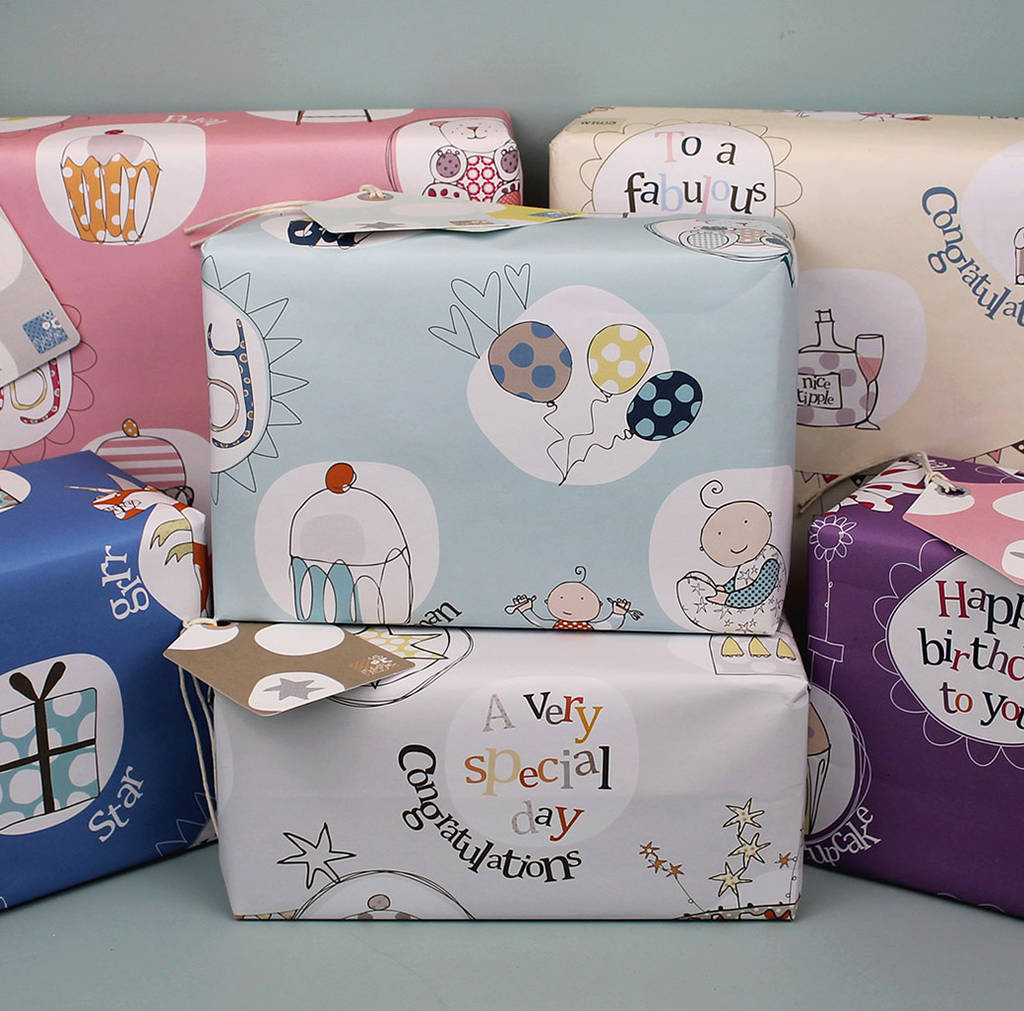In the image, there are six wrapped boxes that appear to be gifts, likely for a child's birthday celebration, possibly a first birthday. Each gift is adorned in charming, sketchy-style wrapping paper featuring a variety of soft colors including pink, pale yellow, pale blue, white, purple, and blue. The designs on the wrapping paper are quite delightful, with playful illustrations of cupcakes, polka-dotted balloons, stars, and adorable babies with a single curly hair in pajamas.

The gift wrap includes various texts such as “Happy Birthday to You,” “A Very Special Day,” “Congratulations,” and partially obscured phrases like “To a Fabulous [something].” One prominent wrap in the lower left corner is particularly blue and says “Star.” The attention to detail in the wrapping is evident, showcasing the same artistic style across all packages, suggesting they might be crafted by the same artist. Additionally, some of the boxes have name tags attached.